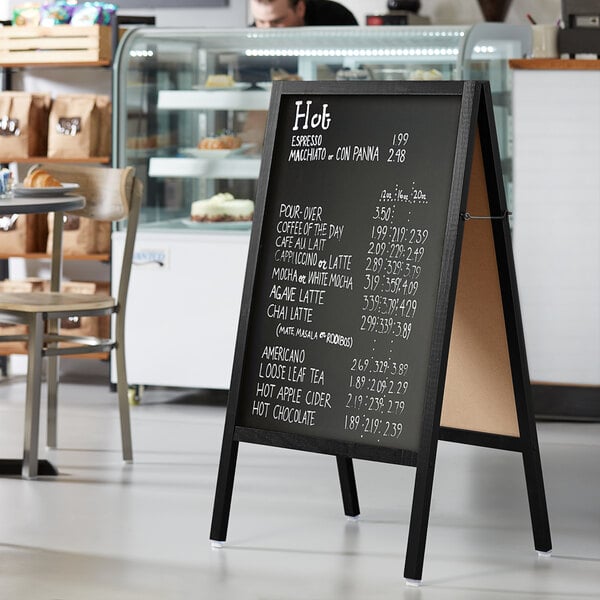In this brightly lit and clean coffee house, an indoor photograph captures a triangular chalkboard menu signboard, set within a black wood-painted frame, positioned prominently on the shiny, light green floor. The black board displays an array of coffee options and prices meticulously written in white chalk. The menu lists items such as Hot Espresso for $1.99, Macchiato or Campagna for $2.48, and various others including Pour Over, Coffee of the Day, Cafe a Latte, Cappuccino or Latte, Mocha or White Mocha, Agave Latte, and Chai Latte, with a variety of prices next to each. To the left of the board, there is a partially visible table and chair, while in the background, a man stands behind a counter looking into a transparent display case, which appears to showcase little cheesecakes and other delectable pastries. The overall ambiance of the coffee house is enhanced by the light streaming in from a window or door on the left, illuminating the white counters and creating a welcoming atmosphere.